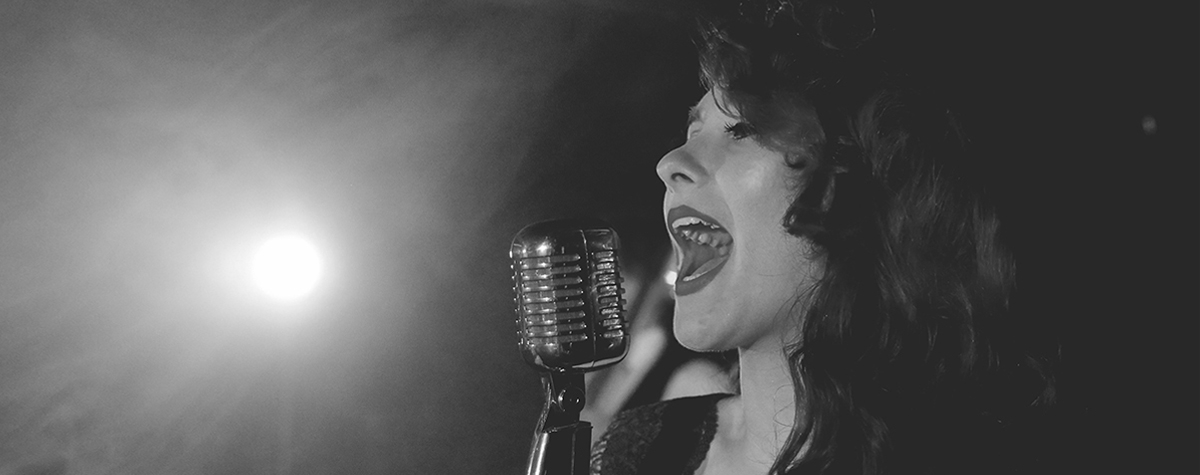In a striking black and white photograph, a woman passionately sings into an old-style, metallic silver microphone. Her long, wavy hair cascades down, almost blending into the dark right side of the image. Her mouth is wide open, eyes closed, conveying the intensity and joy of her performance. A powerful, bright spotlight on the left side bathes her in light, highlighting the texture of her dark lace dress, while the right side of the image remains in shadow, creating a dramatic contrast. The background hints at a concert setting, with blurred figures and instruments adding depth. The entire scene captures the singer's energetic and emotional engagement with her music.